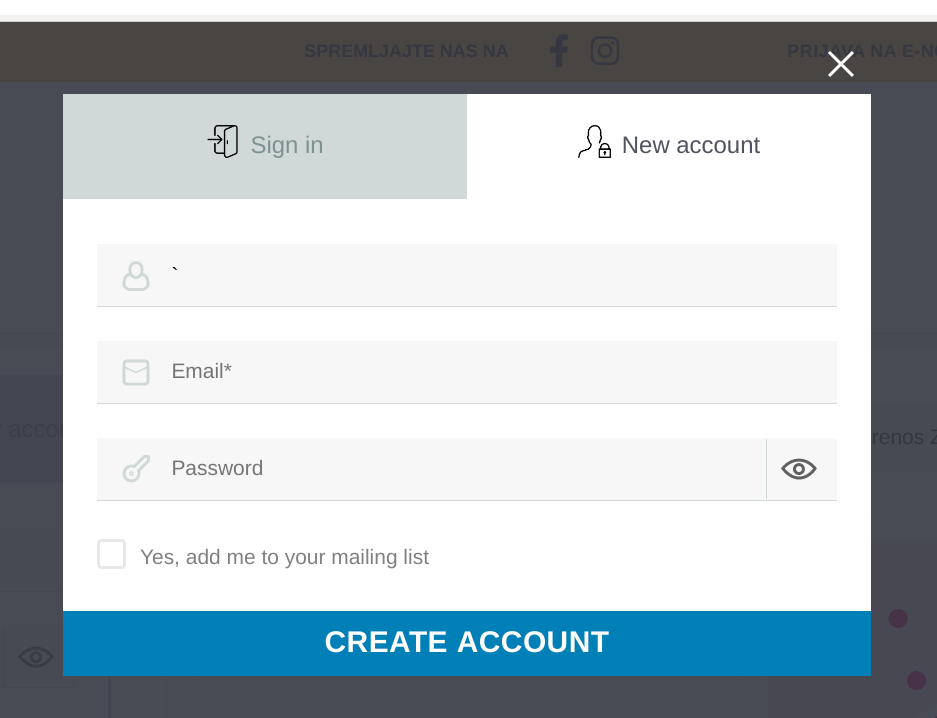The image depicts a screenshot of a sign-up pop-up form, partially obstructing the view of the underlying content and casting dark shadows around the edges. At the top of the form, an illustration resembling an open file folder with an arrow pointing into it is labeled "Sign In." Below this, there's a silhouette of a person accompanied by the text "New Account."

Further down, the form contains various input fields and icons. The first field, which likely prompts for a name, is indicated by a silhouette of a person and is shaded in gray. The next section features a gray envelope icon labeled "Email." Following this, there is a key icon next to the "Password" field, with an eyeball icon located at the end of the line, probably for toggling password visibility.

Toward the bottom of the form, there is a checkbox labeled "Yes, add me to your mailing list." Finally, the form concludes with a teal-colored rectangle containing the text "CREATE ACCOUNT" in white, capital letters.